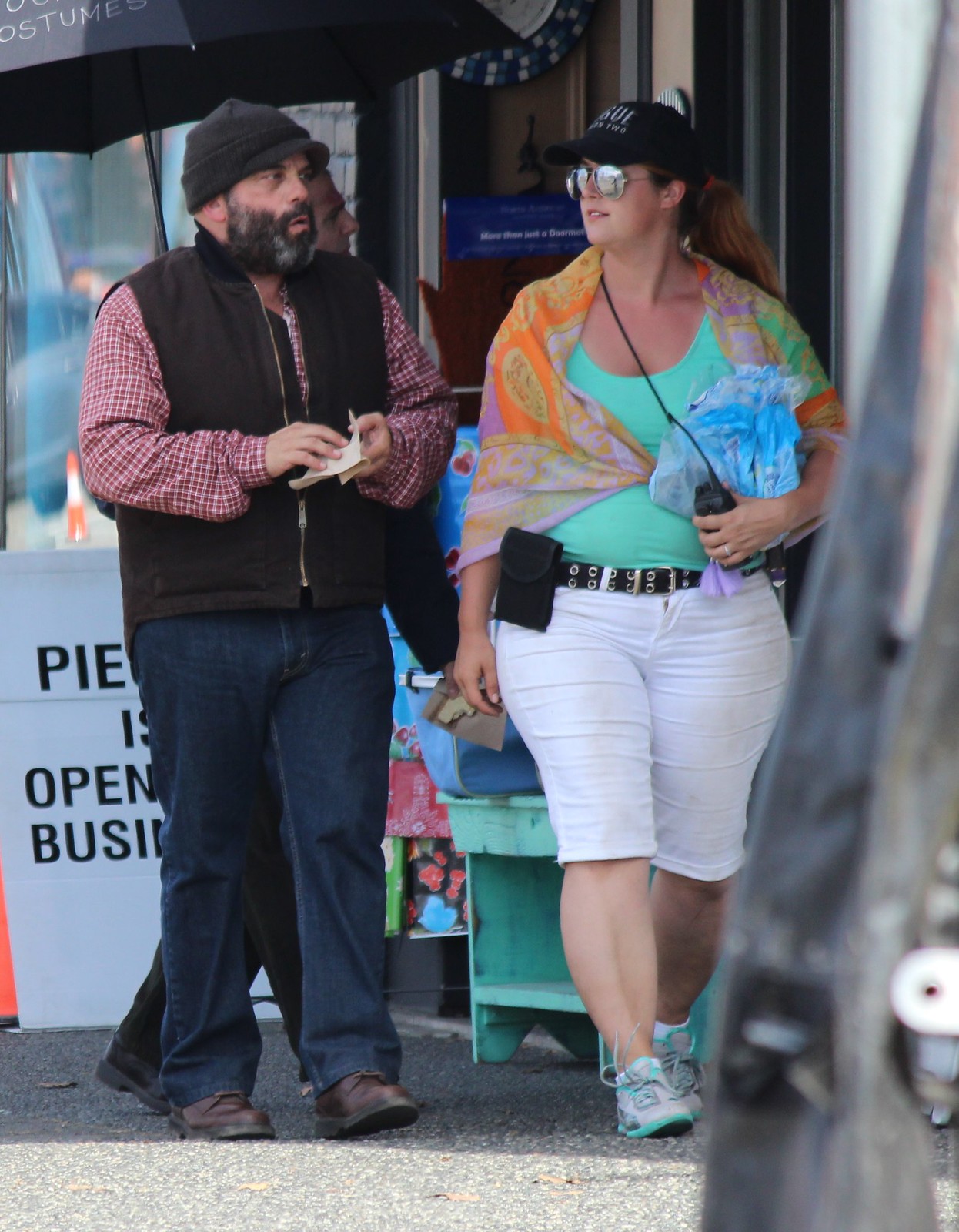The image depicts two people walking down a busy city street, with buildings and businesses in the background. The man on the left, a white man, is wearing blue jeans, brown shoes, a black cap, and a red plaid shirt underneath a brown zip-up vest. He has black and gray facial hair and is holding a piece of paper in his hands. The woman on the right, a white woman, is wearing white Bermuda shorts with a black belt featuring gold grommets, gray and aqua shoes, a turquoise tank top, and a multicolored shawl in shades of orange, yellow, and purple draped over her shoulders. She also wears a black cap with a white print, silver sunglasses, and carries a blue plastic bag slung on her arm. Both individuals are walking on a gray sidewalk, with the man looking at the woman. 

Behind them are various storage bins in colors like turquoise, blue, red, and black. Adjacent to them on the left is a sign partially obscured by their presence, with text mentioning "PIE" and "open for business." Above them in the top-left corner of the image is a black umbrella bearing some text, likely related to a business named "costumes." Additionally, there is a brown door potentially leading into a building. Overall, the scene captures a moment of two people walking amid the hustle and bustle of city life.